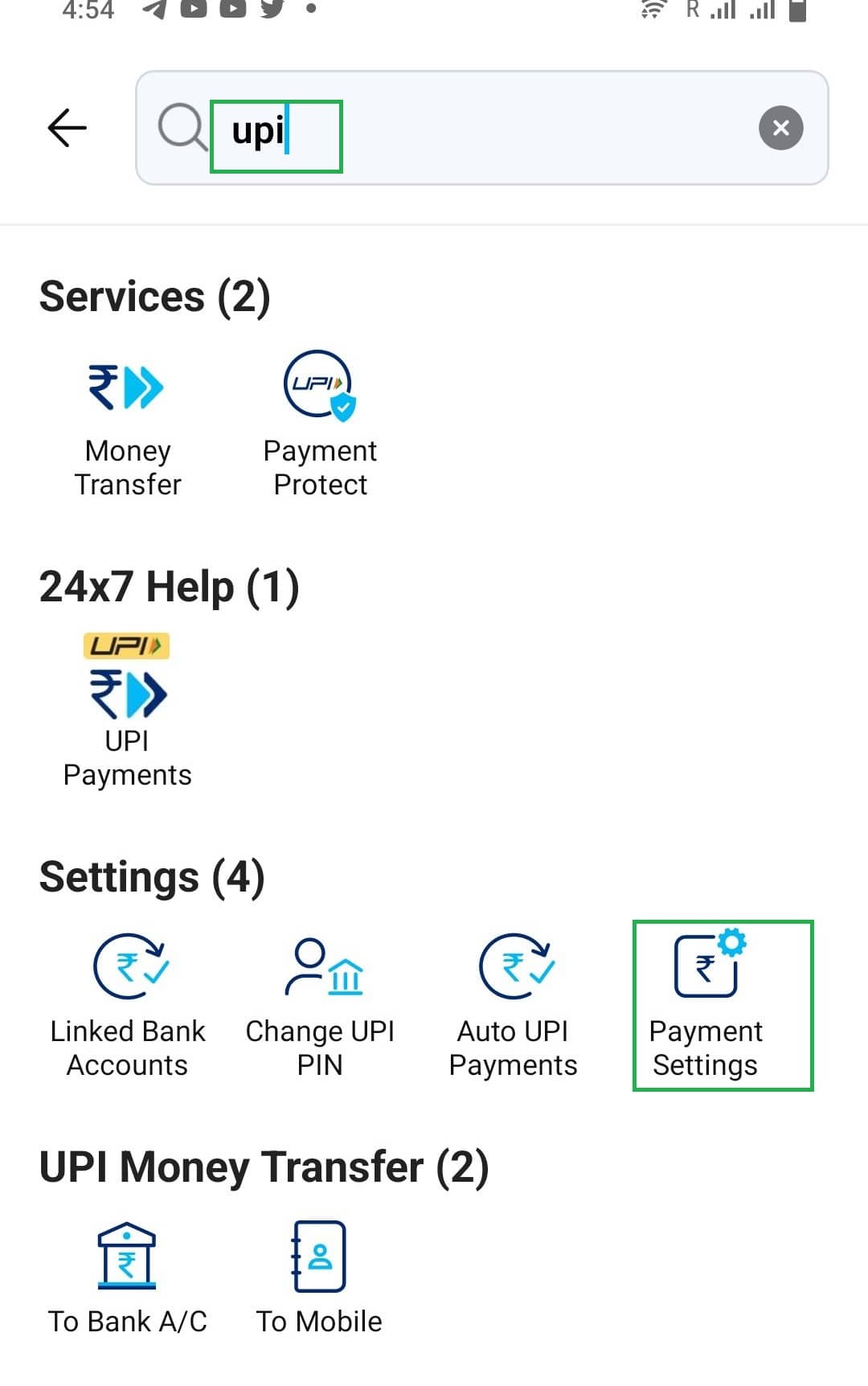The image depicts a smartphone screen displaying a webpage with details about UPI (Unified Payments Interface) services. At the top of the screen, there is a status bar showing a full battery, a strong connection, and the time, which is 4:54 PM. Below the status bar, the search bar prominently features the term "UPI," highlighted with a vertical blue line and enclosed in a green box.

The webpage is categorized under "Services" and lists two main options: "Money Transfer" and "Payment Protect." Additionally, there is a "24/7 Help" section, indicated by a numeral one next to it, suggesting one unread notification or message.

Just above these service listings, there is a small icon, and further down the page, the "Settings" section is denoted with four sub-options: "Linked Bank Accounts," "Change UPI Pin," "Auto UPI Payments," and "Payment Settings," with the latter also highlighted by a green box. 

At the bottom of the screen, the "UPI Money Transfer" section, marked with a numeral two, outlines the transfer options: to a bank account or to a mobile number. Interestingly, there is no company branding or contact information visible on the page, which is unusual for such service-oriented content.